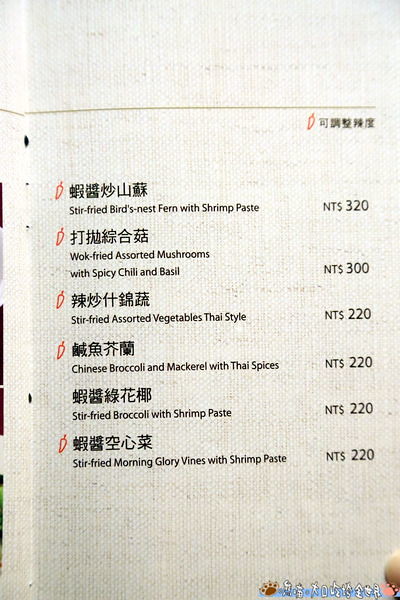The image appears to be the right page of an open menu from a Chinese restaurant, printed on a textured, possibly antique or vintage-style paper. The menu showcases a top margin with a thin yellow line and a logo with Chinese lettering. Each of the six menu items is listed in bold black font, first in Chinese and then in English. The English descriptions of the dishes are: stir-fried bird's nest fern with shrimp paste, wok-fried assorted mushrooms with spicy chili and basil, stir-fried assorted vegetables Thai-style, Chinese broccoli and mackerel with Thai spices, stir-fried broccoli with shrimp paste, and stir-fried morning glory vines with shrimp paste. The prices are listed next to each dish in NT dollars, ranging from NT$220 to NT$320. There is a visible crease on the left side of the page, indicating it is part of an open menu. At the bottom of the image, there is a watermark featuring bear paws on both the left and right sides.